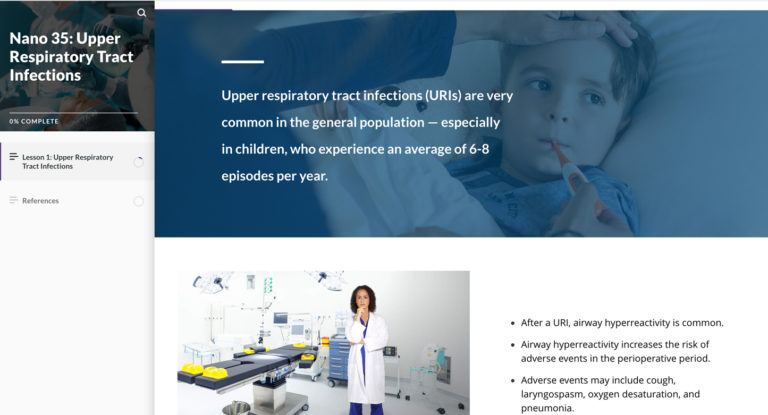The screen capture from the web page features a dual-frame layout.

In the left frame, positioned in the upper left corner, there is a small, somewhat blurry image with white text that reads "Nano 35: Upper Respiratory Tract Infections." Directly below this image, additional text in small black font states, "Lesson Two: Upper Respiratory Tract Infection."

The right frame displays the main content of the web page. At the top of this frame is a poignant image depicting a child with their head resting on a pillow. The child is identifiable by his head and shoulders and is holding a white and red thermometer in his mouth. A caregiver dressed in blue gently places their left hand on the child's forehead while using their right hand to hold the thermometer. Overlaying this image, white text states: "Upper Respiratory Tract Infections. URIs are very common in the general population, especially in children who experience an average of six to eight episodes per year."

This detailed visualization effectively highlights the topic of upper respiratory tract infections, with emphasis on their prevalence in child populations.